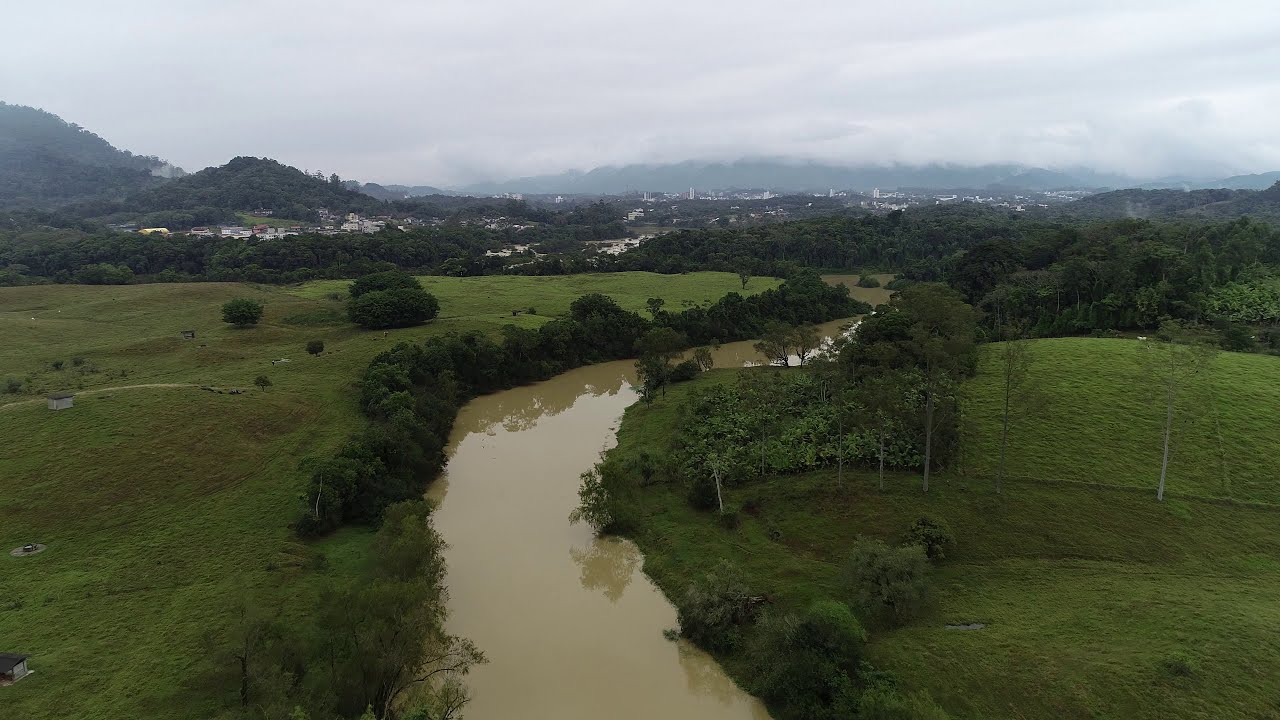The image displays an elevated, detailed view of a swampy landscape taken from approximately 20 to 30 feet above the ground. Dominating the scene is a muddy, brown-tinted river that snakes through the center, starting from the bottom center and bending towards the top right. The river's smooth surface reflects the surrounding lush vegetation. Tall embankments bordered by large, green bushes flank the river, giving way to expansive, slightly hilly grassy fields that extend to the edges of the image. The grass appears muddy and has a brownish hue, suggesting recent rainfall or inherent swampy conditions. In the distance, these fields transition into a forested area and a distant city with small buildings can be seen dispersed among dark mountain peaks. The cloudy sky overhead is a somber gray, indicative of overcast weather.